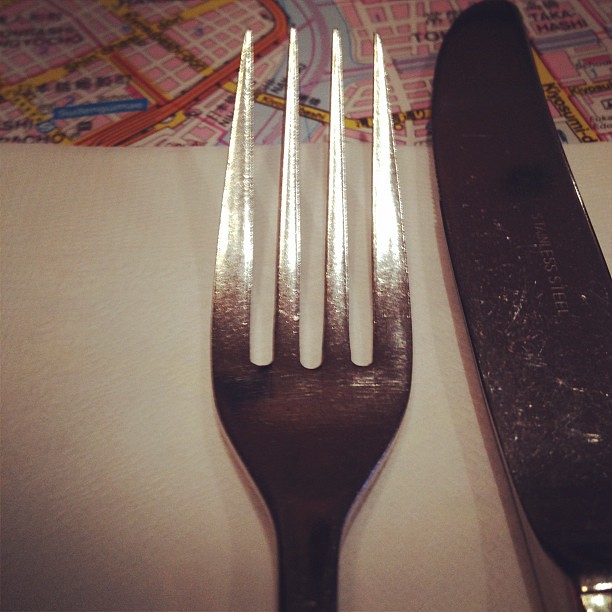This is a detailed close-up photograph of a silver fork and a silver butter knife resting on a white paper towel. The fork, positioned on the left, showcases its tines and neck, while the butter knife, situated to the right, displays its top half. Both utensils exhibit signs of use, including etches and scratches. The butter knife has an inscription that reads "stainless steel," though it's partially obscured by dark tarnished areas, indicating its age and wear. The fork, while not as tarnished, has some wear toward the end of its tines. 

Above the white paper towel, there's a topographical map of a city. This map is richly detailed, with building lots labeled in pink and side roads delineated with white lines. Light blue waterways weave through the city, crossed by bridges in deep pink or purple hues. Black writing is scattered across the map, marking various sections and major streets. Some prominent streets are highlighted in yellow, potentially indicating routes to highways or other bridges. The overall setup suggests an intriguing juxtaposition of everyday objects against a complex urban landscape.